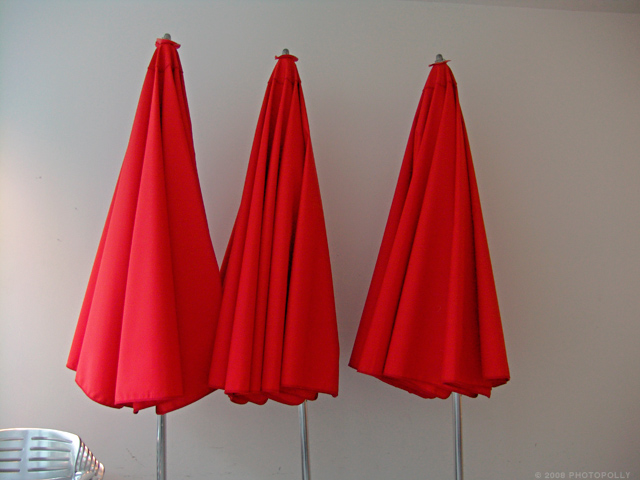The image is a color photograph in a landscape orientation, featuring three bright red closed beach-style umbrellas centered in the frame but slightly leaning more towards the right. Each umbrella stands on a silver metal pole that ends with a silver nub at the top. The two umbrellas on the left are touching, while the one on the right is slightly separated. The pleated red fabric of the umbrellas hangs down, accentuating their closed state. The background is a light faded pinkish-salmon-colored wall, adding a soft contrast to the vibrant red umbrellas. In the bottom left corner of the image, there is a cropped metallic object with horizontal vents, though partially out of view and indistinct. In the very bottom right corner of the photograph, there is a small, nearly illegible white copyright logo followed by the year 2008 and the word "photopoly."